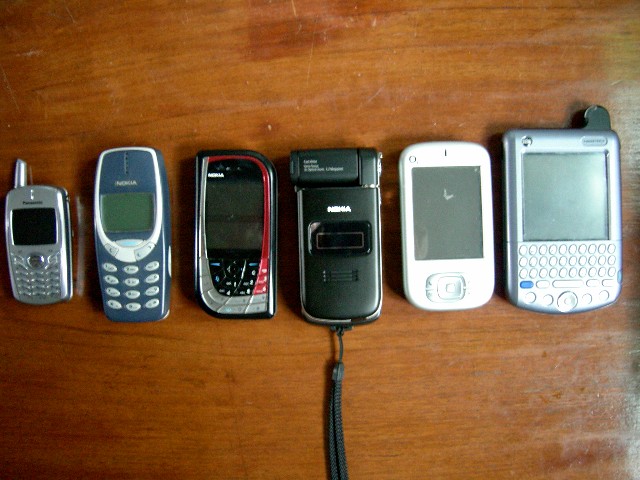Captured from above, this color photograph depicts six vintage cell phones arranged horizontally on a light cherry wood tabletop. From left to right, the phones appear to showcase the evolution of mobile technology, though they remain relics compared to today's standards. 

The first phone is a small, silver Panasonic model with a tiny antenna and keypad. Next is a dark blue Nokia phone with silver accents and a green LCD screen, featuring white navigational buttons. The third phone in line is a Motorola, distinguished by its red and silver casing, a cracked screen, and a mix of black and red buttons.

The fourth cell phone is a black flip phone, possibly another Nokia, with a small central LCD screen and a wrist strap for added convenience. Moving along, the fifth phone is white with a notably larger screen and a single button at the bottom, indicative of the era's shift towards more display-focused designs. The final phone on the right resembles a BlackBerry, characterized by its silver body, expansive screen, and a full QWERTY keyboard in white with two blue function buttons.

Each device, weathered with use, offers a tangible glimpse into the history of mobile communication technology.